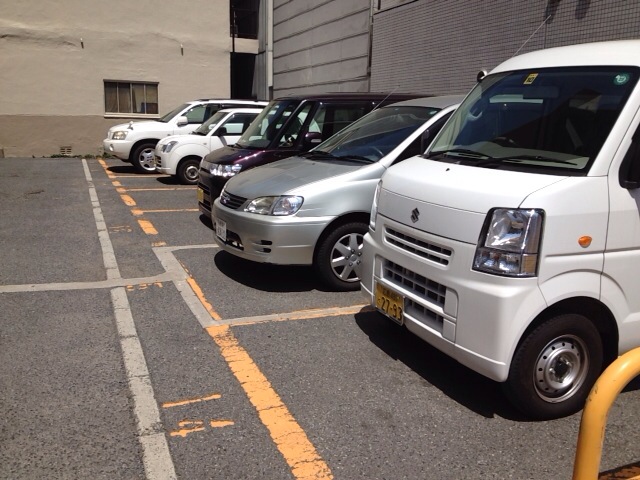This is a detailed photograph of a parking lot situated in a commercial and possibly residential area, likely in Europe or Asia, based on the style of the foreign license plates. The lot has five vehicles, all backed into their parking spaces, which are outlined in yellow lines with orange numbers. The visible spaces are numbered from 10 to 14. The surface is gray macadam with gray and orange stripes. The vehicles, from left to right, are: a sizable white van with a golden license plate reading "27-93", a silver car, a maroon or purple smaller van, a compact white car, and a white small SUV. The parking lot is flanked by taller buildings, creating an L-shape around the lot, including a light tan building on the left and a grayer building to the right, with one building displaying a window with a latch. The scene is sunlit, emphasizing the neat arrangement and urban setting.